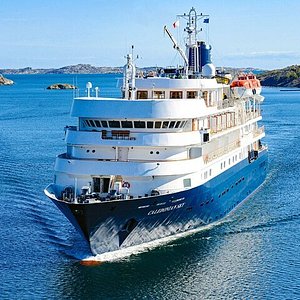The photograph captures a majestic, multi-deck boat advancing towards the camera, situated in the middle of a large, blue body of water with mountains visible in the far background. The boat’s lower section is painted a deep blue, while the top five decks are white and adorned with railings. On the very top, above the bridge, a silver antenna and crane are noticeable, along with orange and white life vests mounted on the highest deck. Although the boat’s name in white text on the nose is indiscernible due to focus issues, distinct elements like windows, balconies on at least three levels, and the impressive wake it produces as it moves through the water are visible. The sky above features a few wispy clouds, further highlighting the serene, daytime outdoor setting.